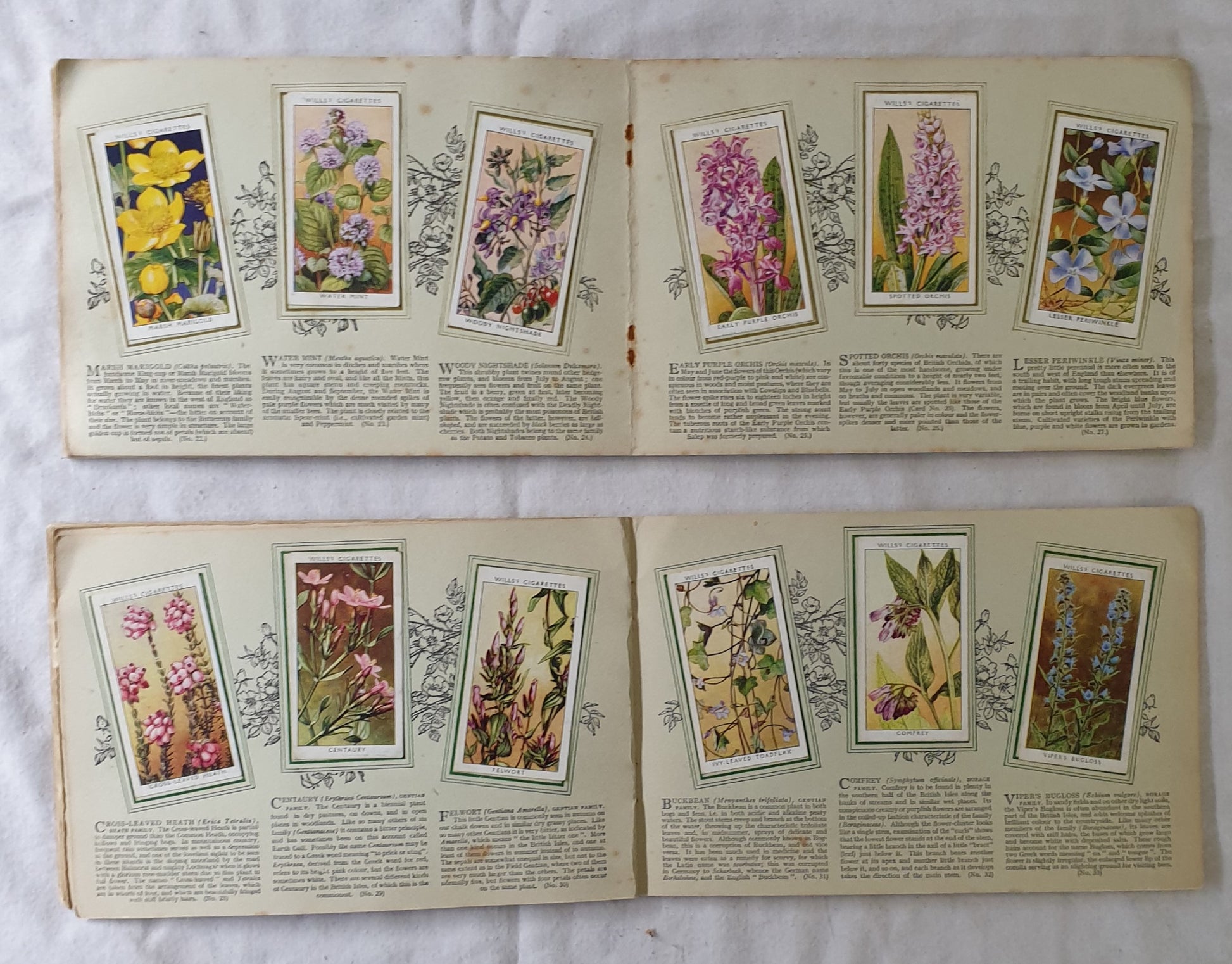The image displays two large, open books, stacked vertically against a white fabric background. Both books are of similar size and appear to be part of the same volume or series, characterized by their long rectangular shape and aged, cream-colored pages. The pages are held together by staples along the spine, which have rusted over time. Each page features detailed color illustrations of various flowers, resembling beautiful watercolor trading cards, with each illustration accompanied by a descriptive paragraph of text in black. On the top book, the left page showcases a yellow flower with yellow petals and a yellow bulb, while the right side features a purple flower. Additional illustrations in the top book include dark purple flowers and light blue flowers. Meanwhile, the bottom book displays different pink flowers on the left page, and a combination of blue and dark pink-purple flowers on the right page, reflecting its purpose as a meticulously illustrated flower catalog.